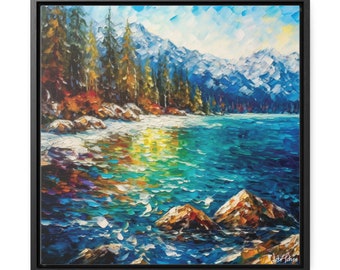The image depicts an exquisitely framed canvas showcasing a post-impressionist landscape painting teeming with vibrant, expressive brushstrokes. The scene captures a tranquil, wintry landscape with a prominent body of water, likely a river or stream, filled with multi-colored reflections of dark, light blue, aqua, yellow, and brown hues. In the foreground, the water is interspersed with large rocks, their surfaces breaking through the waves. The shore in the middle ground reveals a snowy, sandy bank adorned with reddish, orange, and greenish-brown pine trees. Fall colors of oranges, yellows, reds, and whites blend harmoniously amidst the trees, evoking a rich tapestry of autumn. In the far background, the landscape is framed by majestic, snow-capped mountains under a sky with patches of blue and white, diffused clouds. Overall, the painting uses bold, textured brushstrokes to convey movement and reflection, creating a deeply calming and unified natural scene reminiscent of Van Gogh’s style.